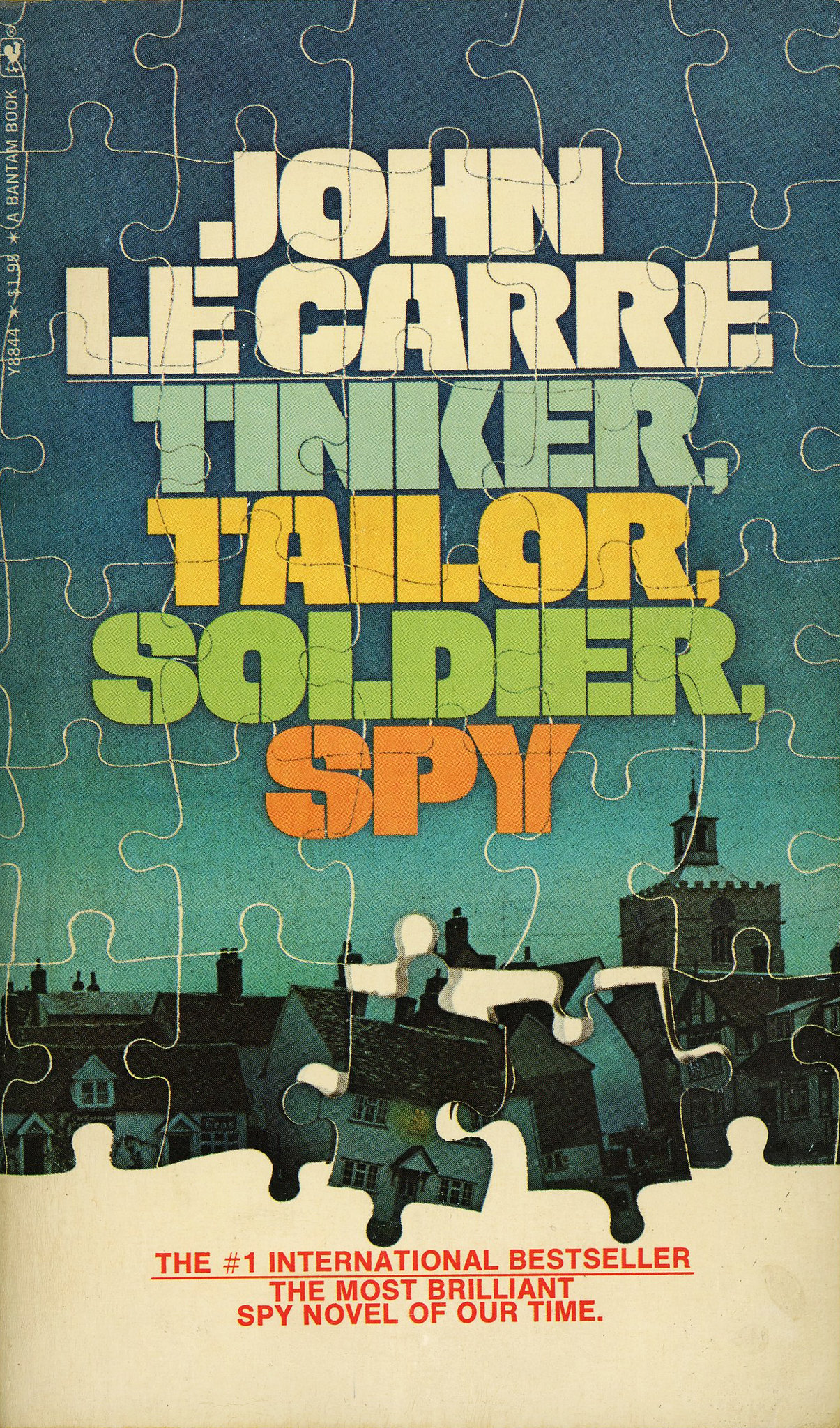The photograph of the book cover presents a highly detailed and evocative image. Dominating the cover is a European-style old-fashioned town, characterized by numerous white-painted, two-story houses with gray roofs, and a prominent castle tower rising in the background. This picturesque townscape is visually broken into several jigsaw puzzle pieces, adding a layer of intrigue and complexity. Above the fragmented city skyline, a vibrant blue sky serves as the backdrop for the bold text: "John le Carré" in white, followed by the title words "Tinker" in blue, "Tailor" in yellow, "Soldier" in green, and "Spy" in orange. The lower section of the cover features a plain white banner, decorated with red outlines mimicking the jigsaw pieces above. Within this banner, the red text proclaims, "the number one international bestseller, the most brilliant spy novel of our time." This design masterfully blends elements of mystery and sophistication, capturing the essence of the iconic spy novel.